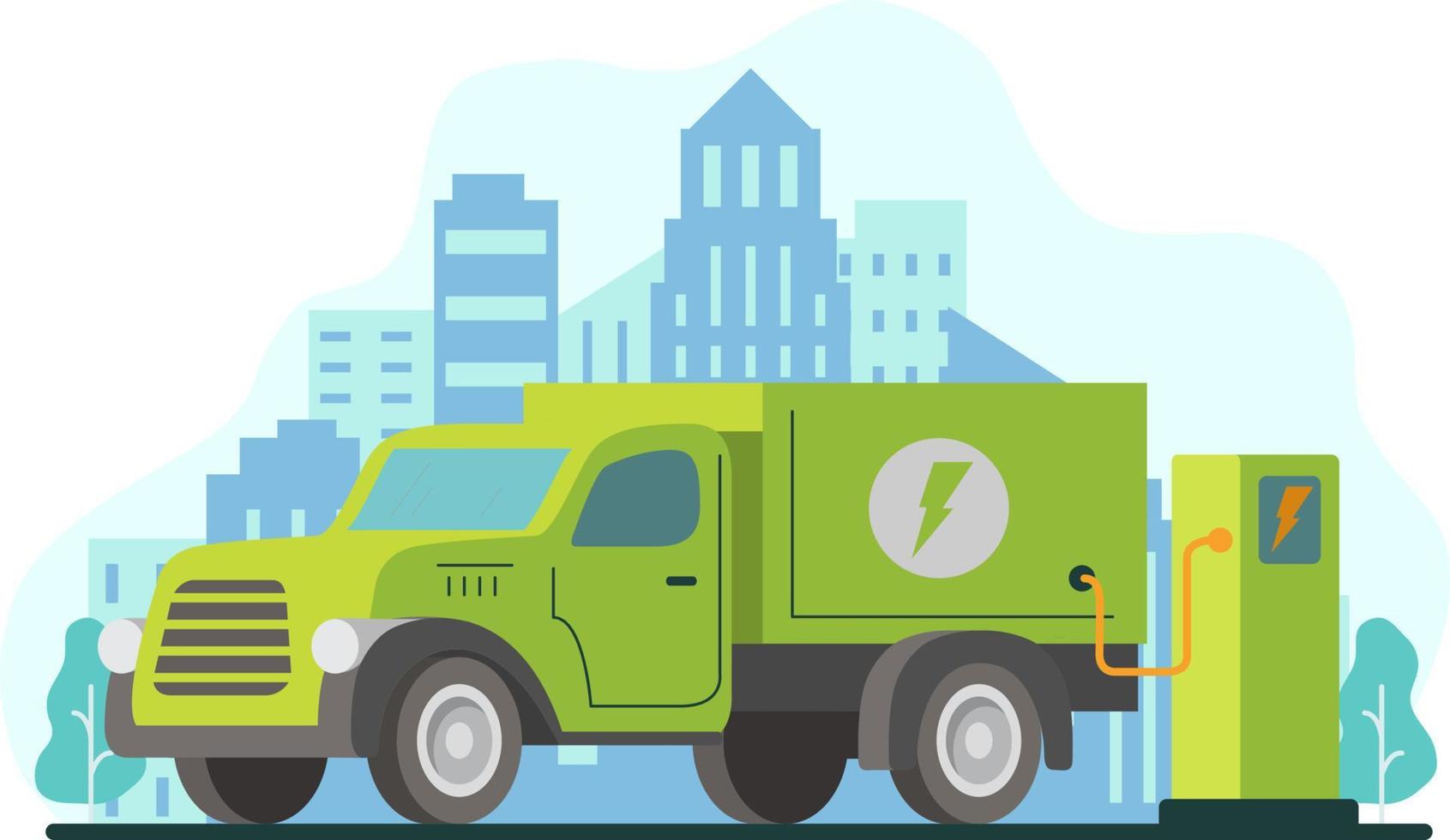The image is a detailed graphical design of a green utility truck hooked up to an electrical charging station. The truck, predominantly green with a gray lower section and wheels, features blue windows and a prominent lightning bolt symbol within a white circle on its side, indicating its electric nature. The charging station, also green, is rectangular and includes an orange charging cable and an orange lightning bolt symbol, complementing the truck's energy theme. Both elements are set against a pristine white background, with a backdrop of a stylized blue cityscape featuring skyscrapers. Additionally, there are trees visible on either side, enhancing the urban environment depicted in the graphic.